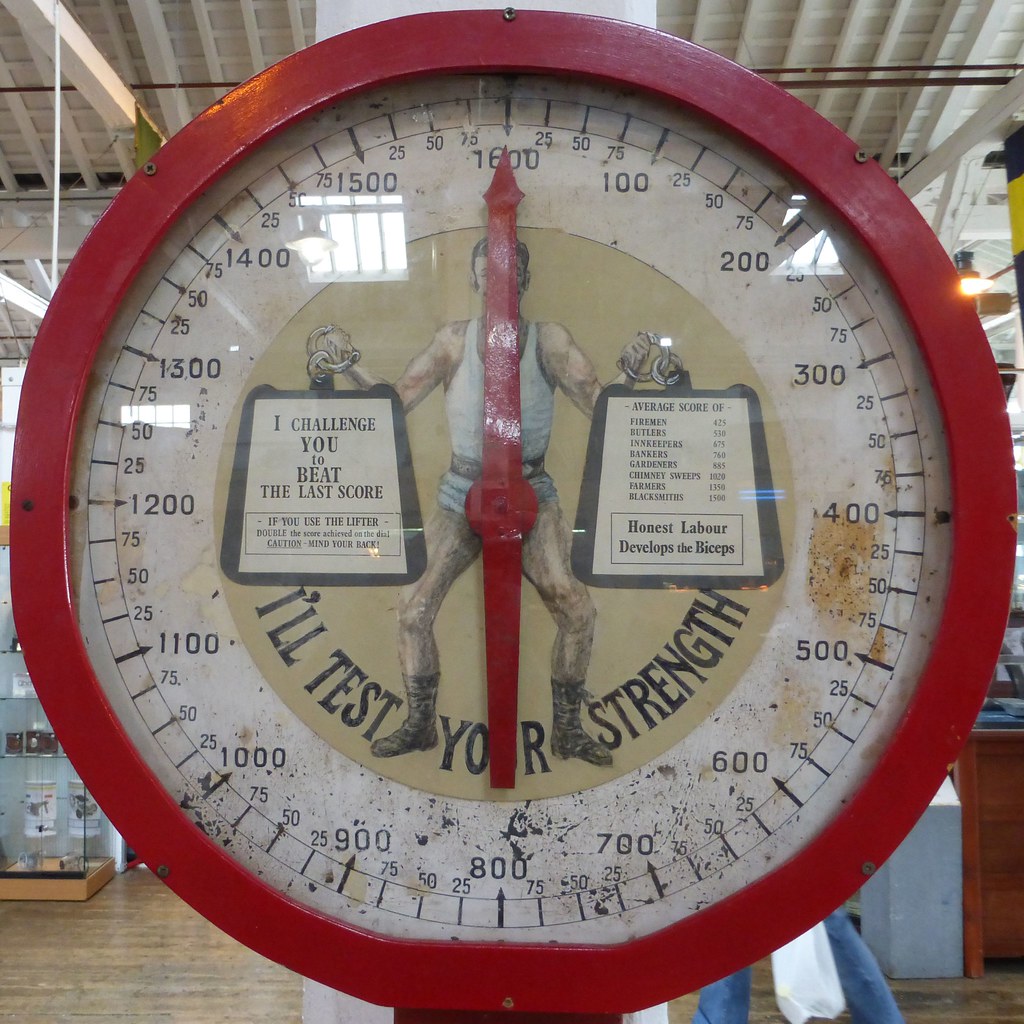The image showcases a vibrant, retro-style analog measuring device, resembling a scale. The device features a bright red frame and a glass-covered face adorned with hash marks and numerical symbols arranged around the circular perimeter. A prominent red needle points upwards to the highest mark on the dial. At the center, set against a white background, is a tan circle displaying an illustration of a muscular man. The man, clothed in a white tank top, shorts, and boots, is depicted holding two large weights, each framed in dark gray with inscrutable black text on a white background inside them. His face is partially obscured by the central red needle. Below the figure, in curved black lettering, is the phrase, "I'll test your strength."

Additional text within the image reads, "I challenge you to beat the last score. If you use the lifter, double the score achieved on the dial. Caution, mind your back." The scale's numerical gradations increase in increments—100, 200, 300—up to a maximum of 1600 and include comparative scores like "firemen 425, butlers 530, innkeepers 675, bankers 760, gardeners 885, chimney sweeps 1020, farmers 1350, blacksmiths 1500," along with the encouraging message, "honest labor develops biceps."

The entirety of this striking device is set against the backdrop of a high-ceilinged, strut-framed building, completing the photograph's unique and detailed composition.